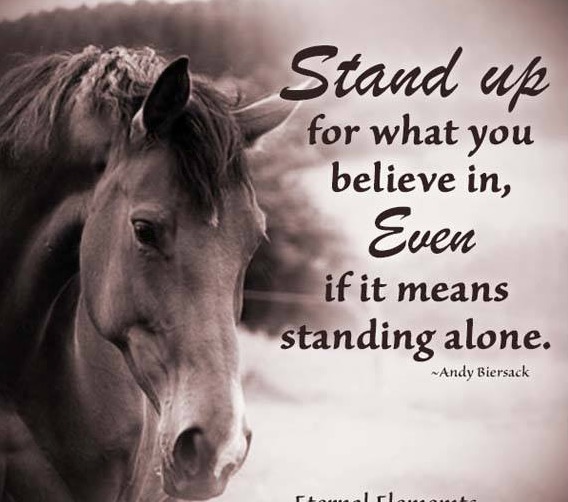The digital image appears to have been created in a program like Photoshop and features a monochromatic, possibly reddish or brownish, hue. On the left side, it displays a close-up of a horse's head with a noticeable white spot on its nose, looking somewhat downcast. The right side of the image fades into white. Overlaying this scene is a motivational quote in dark letters, reading: "Stand up for what you believe in, even if it means standing alone," attributed to Andy Biersack. The text, which shows signs of compression artifacts, is predominantly dark red or wine-colored. Below the quote, a tilde symbol precedes the attribution. Additional text is present at the bottom but is partially cut off and unreadable due to image cropping.